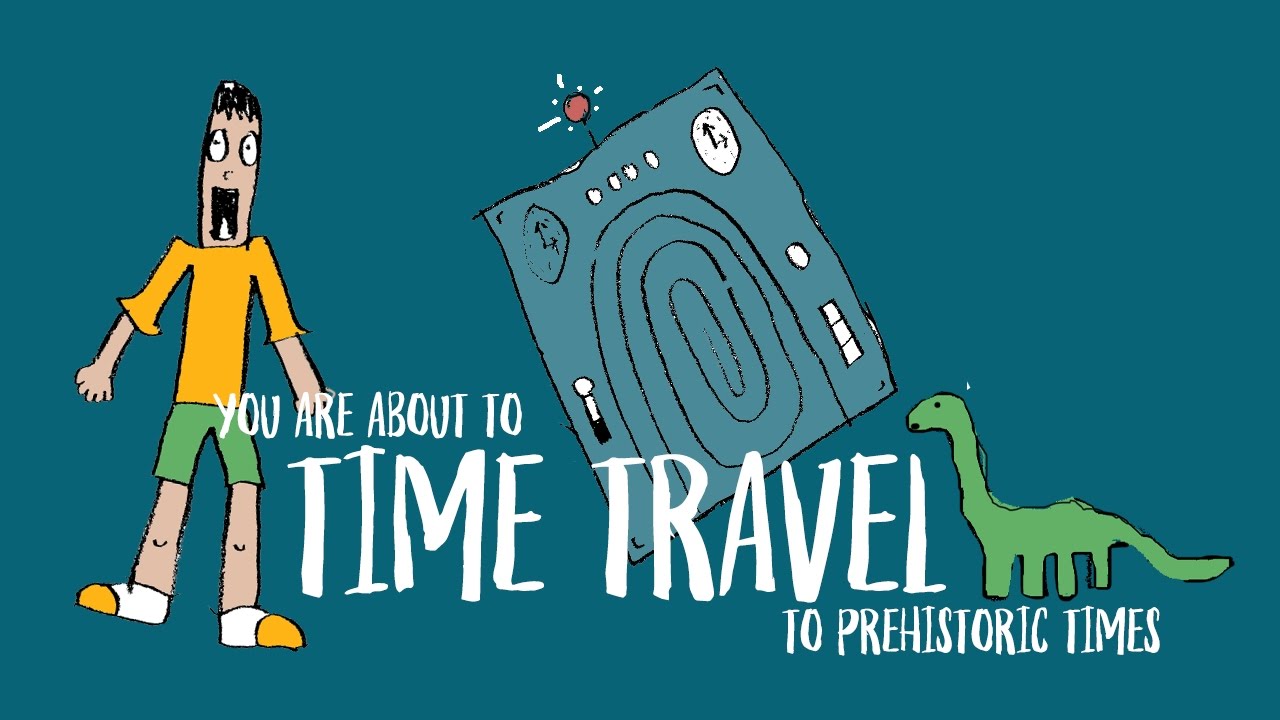The image is a digital cartoon drawing set against a deep blue background, featuring three main elements: a man, a dinosaur, and a scientific contraption. On the left side, there is an animated figure of a man with exaggerated features such as a long face, wide-open mouth, big round white eyes, short black hair, and an elongated, thin body. He is dressed in a yellow t-shirt, green shorts, and white-and-yellow shoes. In the center of the image stands a door-like scientific contraption that appears to be a time machine. This device has a handle on the side, two clock-like dials at the top, and a red ball on top with lines suggesting it emits light or sound. Flanking the time machine on the right is a green dinosaur, possibly a brontosaurus or apatosaurus. The text on the image, with the words "time" and "travel" emphasized in larger font, reads: "You are about to time travel to prehistoric times."